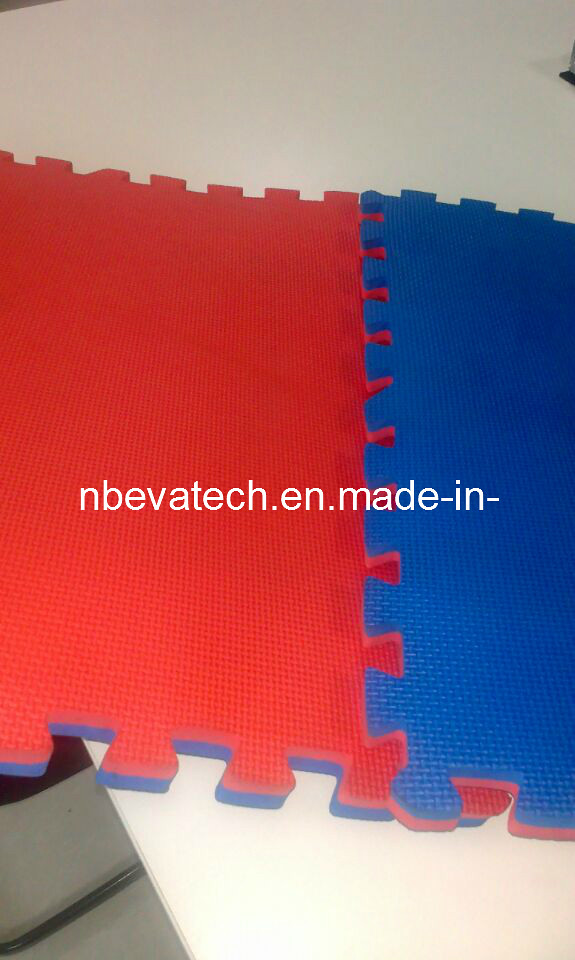This is a detailed image of two large, interlocking foam playmats typically used in children's play areas to provide a soft surface. The playmats are square-shaped with serrated, puzzle-like edges that allow them to connect. The mat on the left is primarily red with a blue border, while the mat on the right is blue with a red border. Both mats have a bumpy texture on the surface. They are placed on a white table, which itself rests on a gray platform. In the middle of the image, a part of a URL, "n-b-e-v-a-tech dot e-n period made hyphen in hyphen," is visible in white font.